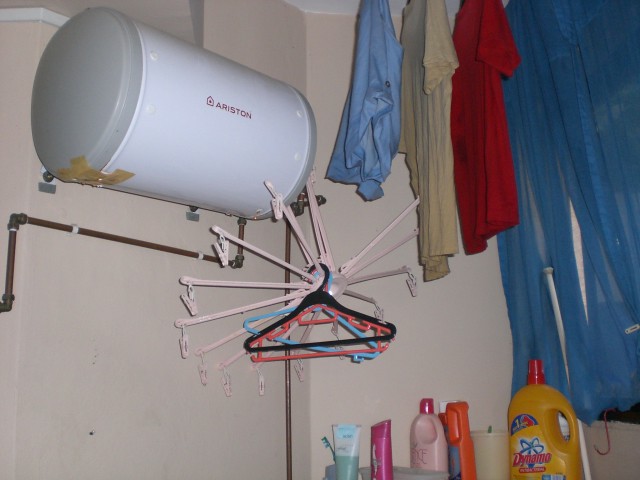This low-quality color snapshot photograph captures the cluttered ambiance of a laundry room. Dominating the left wall is a horizontally-mounted white cylindrical water heater with gray capped ends labeled "Ariston," connected by copper pipes, some covered with masking tape. Hanging from near the ceiling are garments: a blue shirt, a beige shirt, and a red shirt, possibly joined by a curtain or dress. Clothes hang from a unique plastic contraption equipped with radiating arms that extend in a sunburst pattern, each arm adorned with plastic clips for drying clothes. On the right side, various bottles, jars, and tubes—presumably laundry detergents, cleansers, and even some cosmetics—reside along with a toothbrush, hinting at a utilitarian space. The overall scene is dappled with a mix of garments and practical laundry items, underscoring the room’s functional yet disorganized nature.